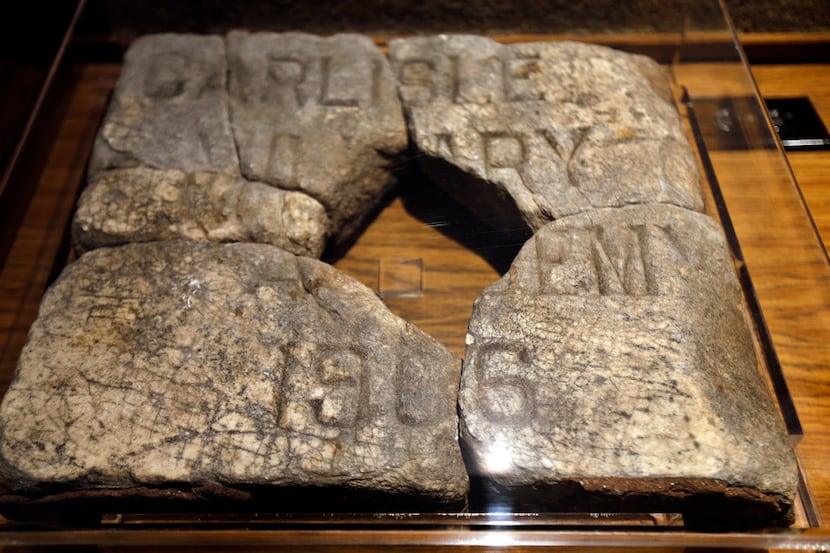The image depicts a broken and dirty engraved stone, possibly made of concrete or selectively stained white, that has been carefully reassembled on a brown wooden platform and encased in a clear plexiglass box for protection. The stone is fragmented into six pieces with a diamond-shaped gap in the middle. The topmost visible engraving reads "Carlisle," and below it is a partially obscured word that appears to end in "ARY," likely suggesting it may refer to a foundry. Further down, the letters "E-M" are visible, hinting it might be part of the word "museum." At the bottom, the clearly visible date "1906" is engraved. The arrangement suggests the stone is of historical significance, akin to a marker, with the missing and broken segments hinting at its aged and weathered past.